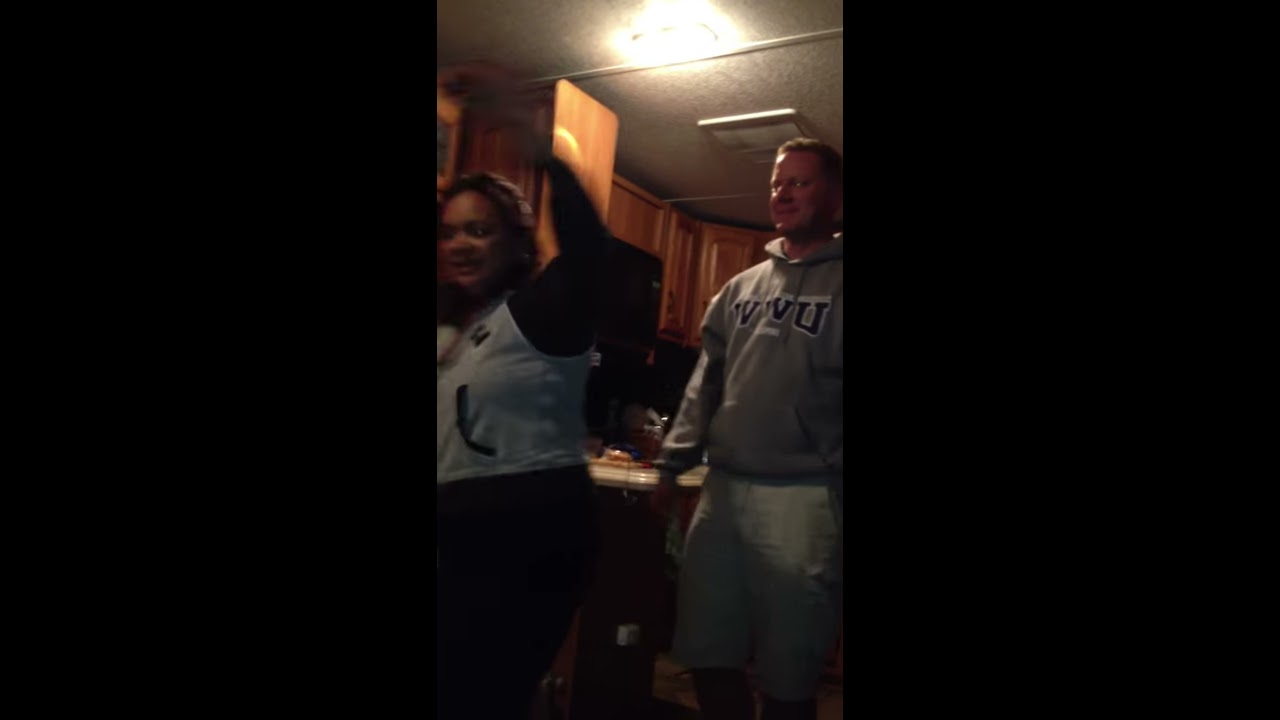This is a horizontally aligned rectangular image with thick black vertical borders on each side, focusing on a narrow vertical, central section where two people are visible. The setting appears to be a kitchen, featuring dark brown cabinetry that doesn't reach the white ceiling, with various items spread across the countertop and a microwave visible beneath the cabinets. The man on the right, a white male with very short hair, is dressed in a gray hoodie with "WVU" printed in blue letters on the chest, and he is wearing khaki-colored shorts. He is smiling at the woman to his left, who has darker skin and shoulder-length brown hair. Although slightly blurred, the woman appears to be in a celebratory pose, possibly dancing, with her left arm raised above her head. She is wearing a white and black top with dark pants. This image captures a lively moment, perhaps from a family gathering, party, or a get-together during a sporting event.